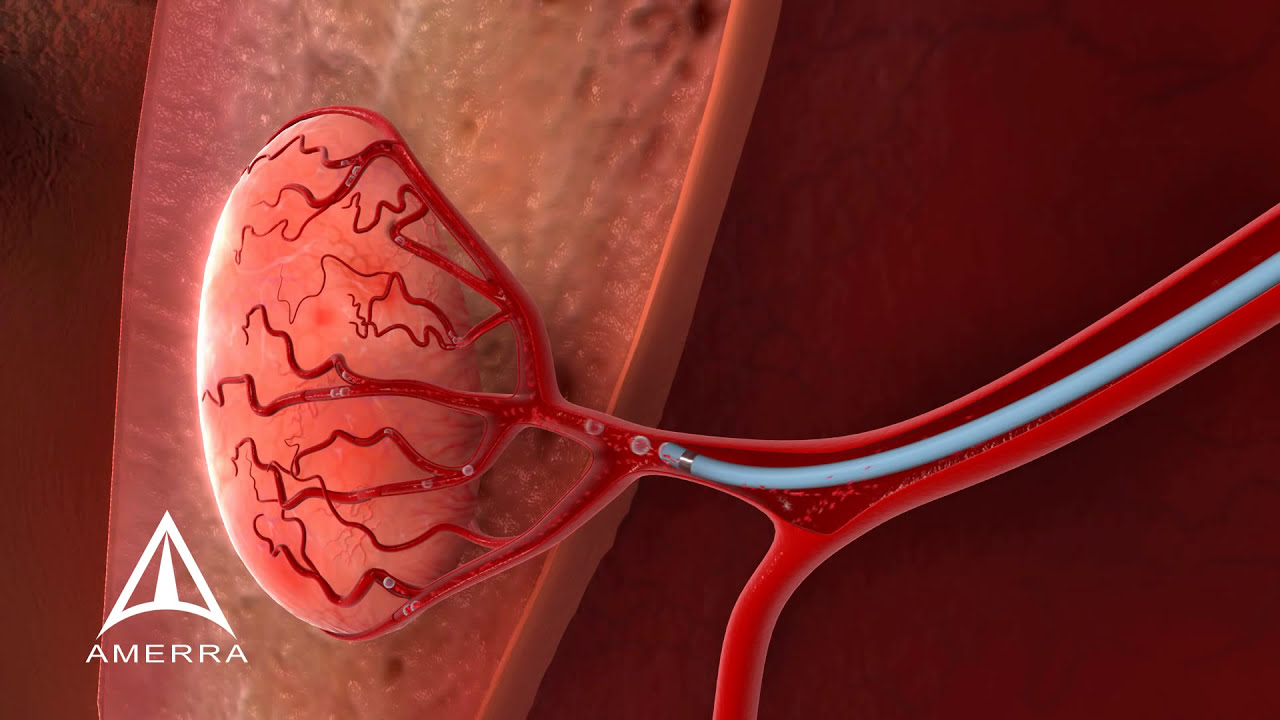This detailed computer-generated diagram depicts a kidney, which is a kidney-shaped, oval pink organ with a multitude of blood vessels attached to it. These smaller vessels converge into a larger red vein that extends to the right side of the image. Within this larger vein, which is sliced open for clarity, there is a long, thin blue tube that appears to have a silver, round collar at one end. This setup suggests an exploratory medical device within the vein. On the bottom left of the image, there is text along with a logo resembling an upside-down V or a triangular insignia, and the word "AMERRA" is displayed, spelled A-M-E-R-R-A.